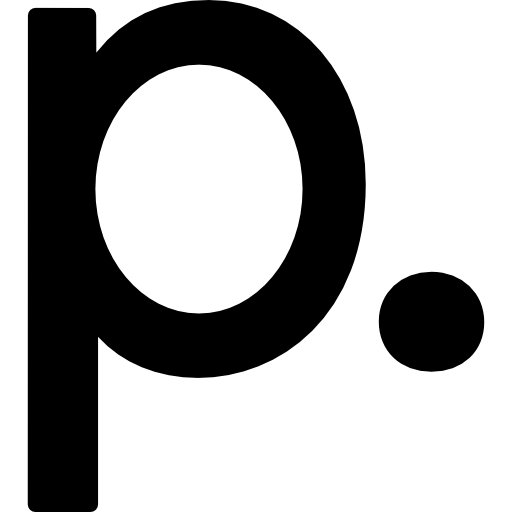The image features a minimalist, computer-generated design set against a solid white background. Dominating the left-hand side is a large, black lowercase letter "p," with the loop of the "p" hollow and white inside. Positioned to the right of the "p" is a medium-sized black dot, aligned at the same vertical level as the loop of the "p." The overall composition is stark and simple, emphasizing the strong contrast between the black elements and the white background. The image is clear and sharply defined, suggesting it may be an abstract or graphic representation.